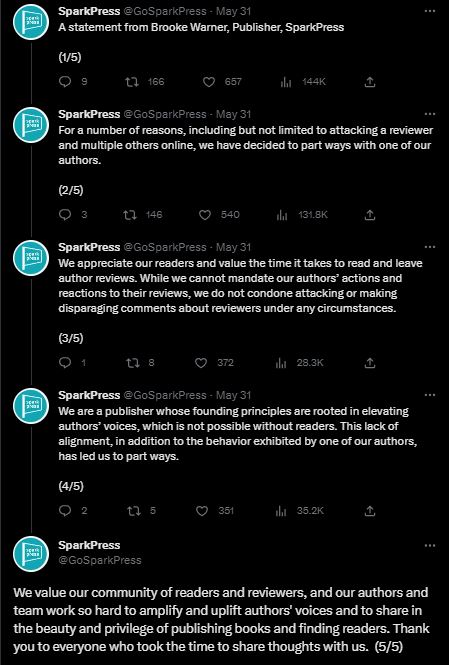A detailed caption for the described image could be:

---

This is a detailed screenshot of a comment chain on the social media platform formerly known as Twitter (now X), originating from the account of Spark Press (@GoatSparkPress) dated May 31st. The series of comments starts with an official statement from Brooke Warner, the publisher of Spark Press.

The chain begins with Spark Press announcing their decision to part ways with one of their authors due to the author's inappropriate behavior online, which included attacking a reviewer and multiple others. The post emphasizes their appreciation for their readers and the value of the time they invest in reading and leaving reviews. Spark Press states their disapproval of any author attacking or making disparaging comments about reviewers under any circumstances.

Visually, the post is presented on a black background with white text. The Spark Press logo, appearing at the top, is a simple design consisting of a green circle featuring a small flag with text inside.

The subsequent comments underscore the publisher's founding principles, which focus on elevating authors' voices. The final comment in the chain reiterates Spark Press's commitment to their community of readers, reviewers, and authors, expressing gratitude to those who shared their thoughts and feedback.

---

This description offers a comprehensive overview while maintaining detail and clarity.